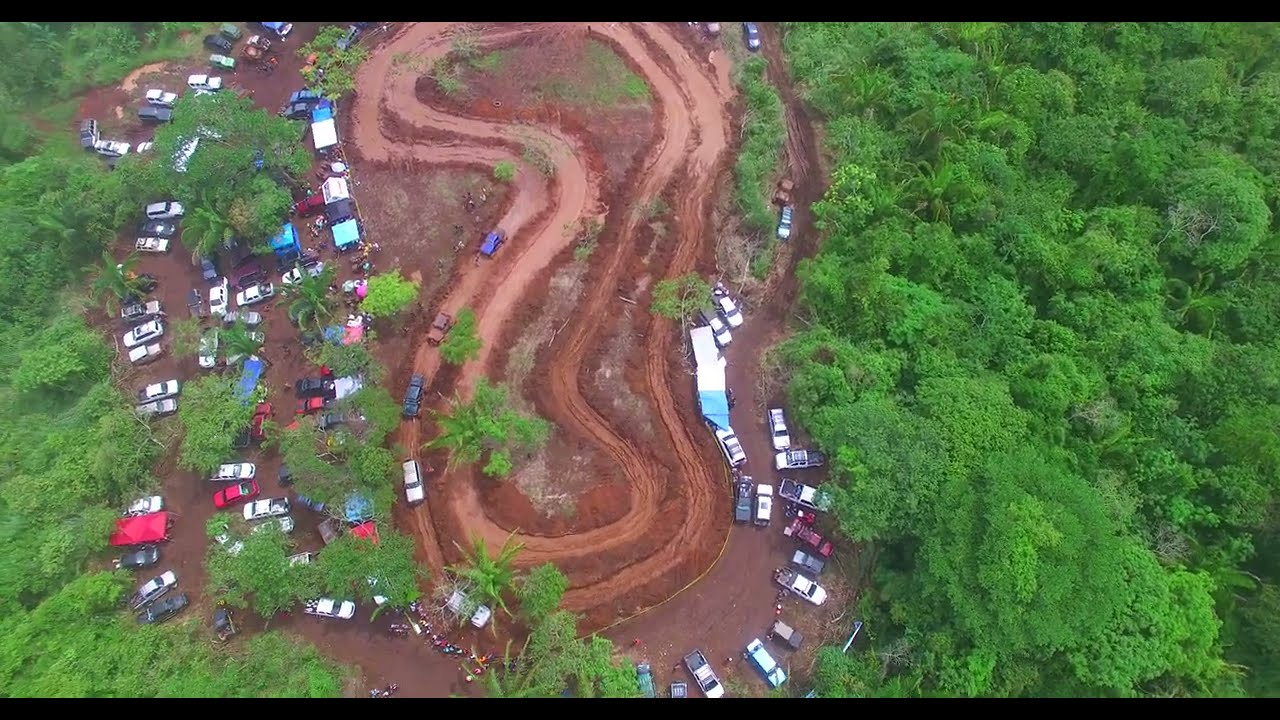This aerial photograph captures a racetrack with a distinctive figure-eight shape, composed of muddy, dirt paths that suggest recent rainfall, though the weather is now clear. Surrounding the track is a lush, subtropical forest with varying shades of green, including lime green and dark green trees. Encircling the racetrack are hundreds of parked vehicles—white cars, pickup trucks, camper vans, and a mix of other colors like red, black, and blue. The racetrack itself features five vehicles driving in a line, navigating the elongated, curving course. The right side of the image is particularly dominated by dense tree canopies, which are viewed from such a height that individual trees blur into a sea of green. The photograph is bordered at the top and bottom with thin black bars, adding a frame to the scene.